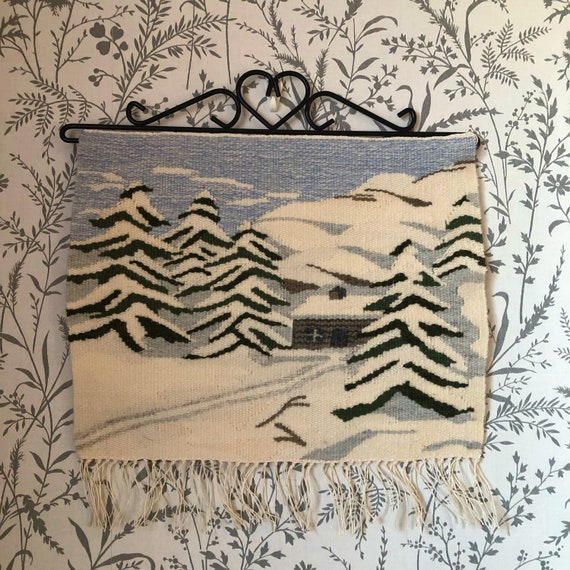The image captures a detailed tapestry-like wall hanging that features a snowy winter scene with a log cabin at its center. The cabin is brown, surrounded by dark forest green evergreen trees laden with white snow on their branches. The snow also blankets the roof of the cabin and the ground. Tracks lead up to the front of the cabin, adding depth to the scene. In the background, the sky is a light blue, contrasting with a snow-covered hill. The wall hanging is adorned with white fringe at the bottom and is suspended by a black hanger. It is displayed on wallpaper with a white background and an intricate pattern of small gray ferns and leaves.